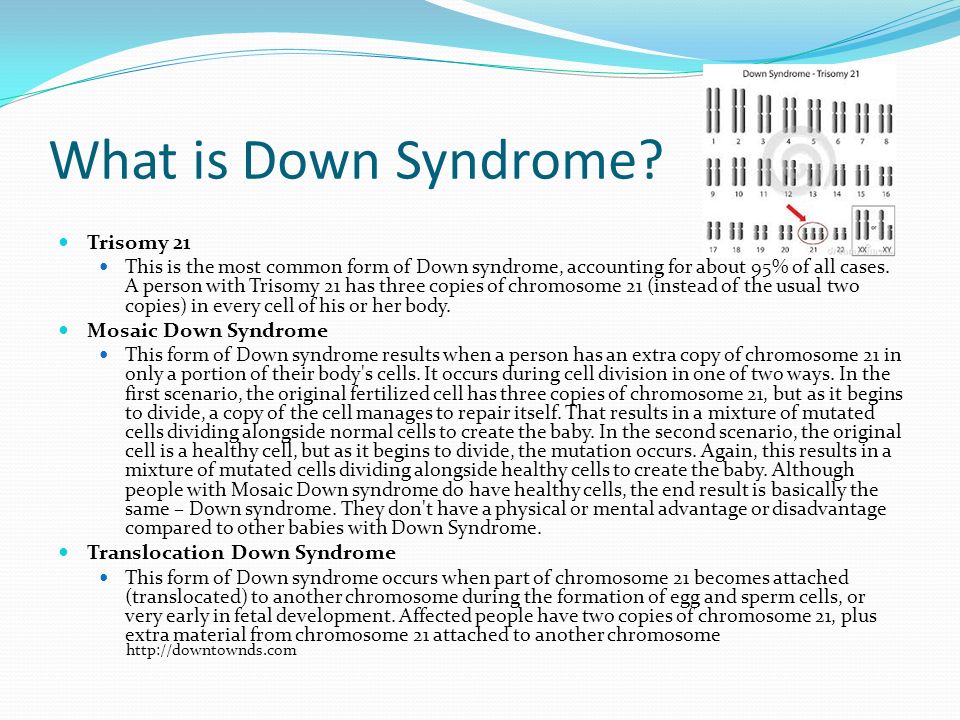This image provides an informative overview of Down syndrome, likely sourced from a pamphlet or a website. The background is primarily white, accentuated at the top by a stylized, abstract wave design in shades of white, turquoise, light blue, dark blue, and grayish blue. 

Dominating the right side, an eye-catching headline in large blue text asks, "What is Down syndrome?" Adjacent to this headline is an inserted image illustrating genetic coding, enhancing the thematic relevance of the content. 

Beneath the headline, three main bullet points are presented:

1. **Trisomy 21**: Marked by a blue bullet point and a bold black heading, this section provides detailed information about the most common form of Down syndrome.
  
2. **Mosaic Down syndrome**: The second bullet point delves into this specific type of Down syndrome, offering pertinent details to distinguish it from other forms.

3. **Translocation Down syndrome**: The third bullet point focuses on this type of Down syndrome, accompanied by a descriptive paragraph.

The image concludes with a website address situated at the bottom: [http://downtownds.com](http://downtownds.com), inviting viewers to seek further information.